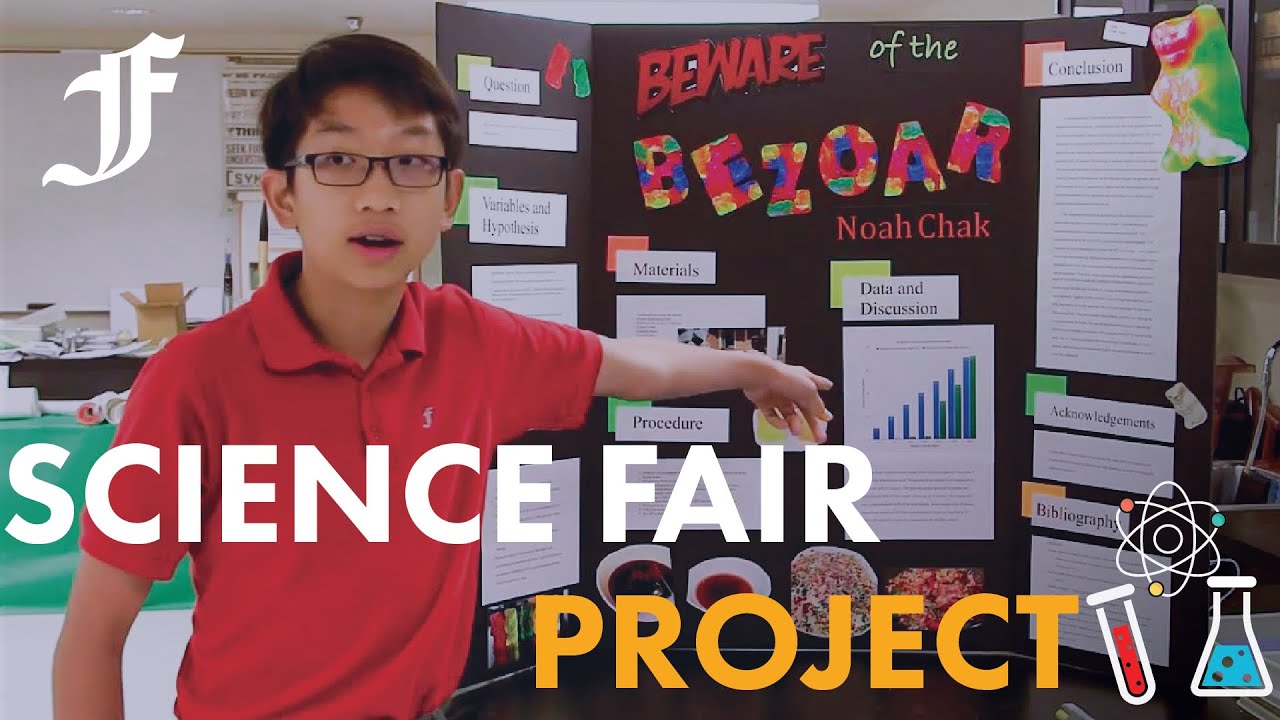In this image, a young adolescent boy named Noah Schock is depicted standing and pointing towards an elaborate display. The display, crafted from a large piece of cardboard painted black, features white papers meticulously pasted or taped to its frame, detailing various pieces of information. Among the colorful lettering, his name "Noah Schock" stands out in vibrant orange. The display's title, "Beware of the Bezoar," is prominently written with "Beware" in a striking combination of red and white, and "Bezoar" spelled out in multicolored letters—red, green, blue, and yellow.

Noah, dressed in a red shirt and sporting black-rimmed glasses, appears engaged with his presentation. Overlaying the photograph in the upper left corner is a prominent letter "F," beneath which the title "Science Fair Project" is displayed in bold white and yellow letters. Accompanying the title are icons of beakers containing blue and red liquids, along with a small atom icon, underscoring the scientific theme of the event.